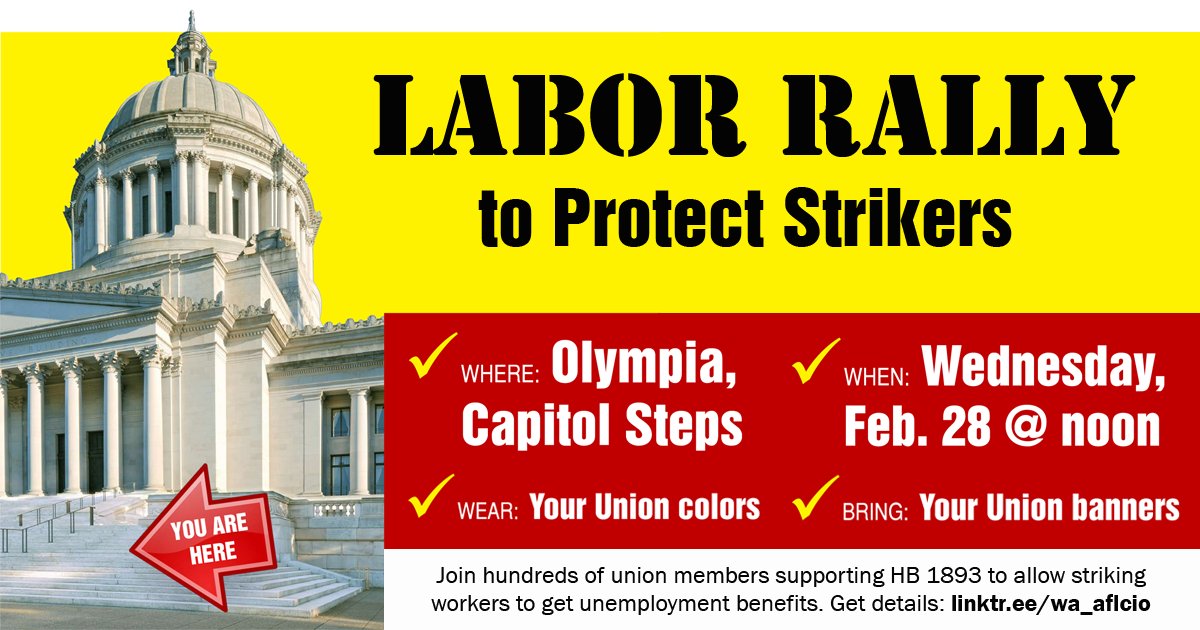The flyer is a detailed and visually organized color advertisement promoting a labor rally. It features a prominent cutout image of the white state Capitol building with its iconic round dome positioned on the left side. A red arrow labeled "You Are Here" points to the Capitol steps. The top of the flyer displays a bold heading in black text on a yellow background that reads, "Labor Rally to Protect Strikers." Below this, a red text box lists essential details in white text alongside yellow checkmarks: 

- "Where: Olympia Capitol Steps"
- "When: Wednesday, February 28 at Noon"
- "Wear: Your Union Colors"
- "Bring: Your Union Banners"

At the bottom right of the flyer, additional black text on a white background urges participants to "Join hundreds of union members supporting HB 1893 to allow striking workers to get unemployment benefits," accompanied by a web address for further details.